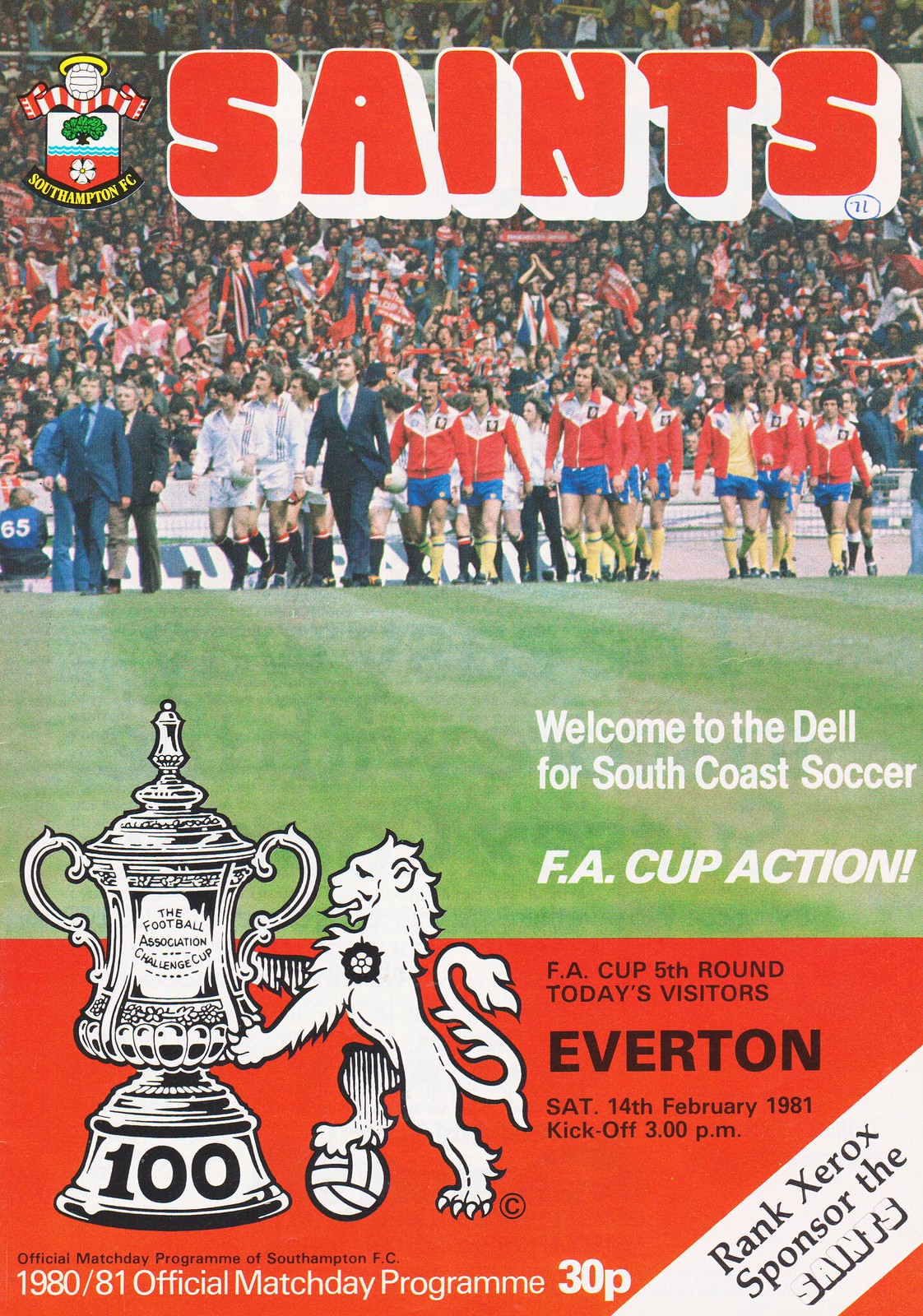This is a vintage football program cover from 1981 showcasing a vibrant scene from a Southampton FC match. Dominating the top, bold red letters with a 3D white border spell out "Saints." To the left, the Southampton FC crest features a flower, water, tree, and a ball with a halo, adding a touch of tradition and pride. Below, white text reads "Welcome to the Dell for South Coast Soccer FA Cup action," setting the stage for the excitement of the FA Cup fifth round match against Everton on Saturday, 14 February 1981, with a kickoff time of 3 p.m. The featured photo captures the Southampton team in classic red and white long-sleeved tops, blue shorts, and yellow socks, standing on a bright green field with a large, cheering crowd waving flags in the background. Men in suits, likely the coaches and managers, add a formal touch to the scene. At the bottom, the program notes it as the "1980 to 81 official matchday program" available for 30 pence, and mentions the sponsor "Rank Xerox". The FA Cup graphic includes a large trophy with a lion's paw resting on a ball, enhancing the historic and competitive nature of the event.